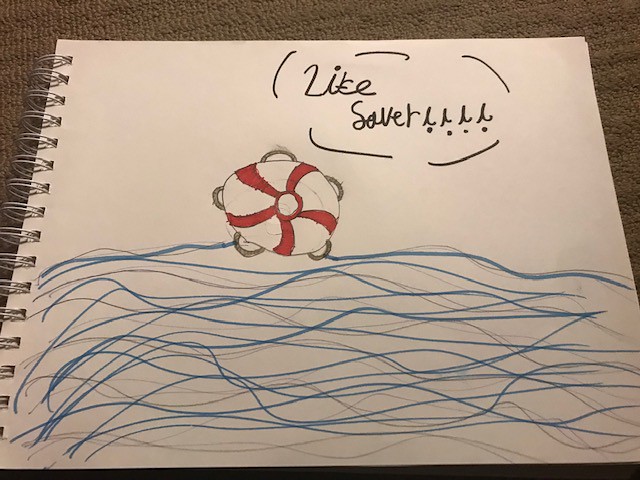The image is a slightly wider-than-tall, top-down view of a wooden table with a rich, textured brown surface featuring roughly horizontal grain lines. Resting on the table is a square, spiral-bound sketchbook, identifiable by its metal double-ring bindings on the left through square punch holes. On the sketchbook's off-white sheet of paper, there's a marker drawing of a circular life preserver, depicted with five red stripes radiating outwards against a white background. This life preserver floats atop a series of blue wavy lines, representing water, drawn in dark and light blue hues. Above the life preserver, towards the right, the text "life saver!!!!" is inscribed, likely in pencil. The background edges of the image reveal a textured carpet or bedspread, adding a plush contrast to the wooden table.